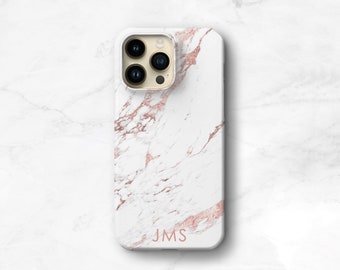This is a detailed product photograph showcasing a marble-textured iPhone case, meticulously staged on a white marble background with gray streaks to draw attention to the case. The phone case itself features a sophisticated design with a white base adorned with elegant pink streaks, mimicking the appearance of polished marble. The precise pink text "JMS" is prominently displayed near the bottom of the case. The top left corner of the case has a square cutout accommodating three black, circular camera lenses, alongside a smaller black dot likely functioning as the camera flash. The rectangular case, longer on the left and right sides than on the top and bottom, appears to be designed for a model such as the iPhone 12 or 14. The seamless coordination between the case and the marble background enhances the visual cohesiveness of the photograph, ensuring the viewer's focus remains steadfast on the product.